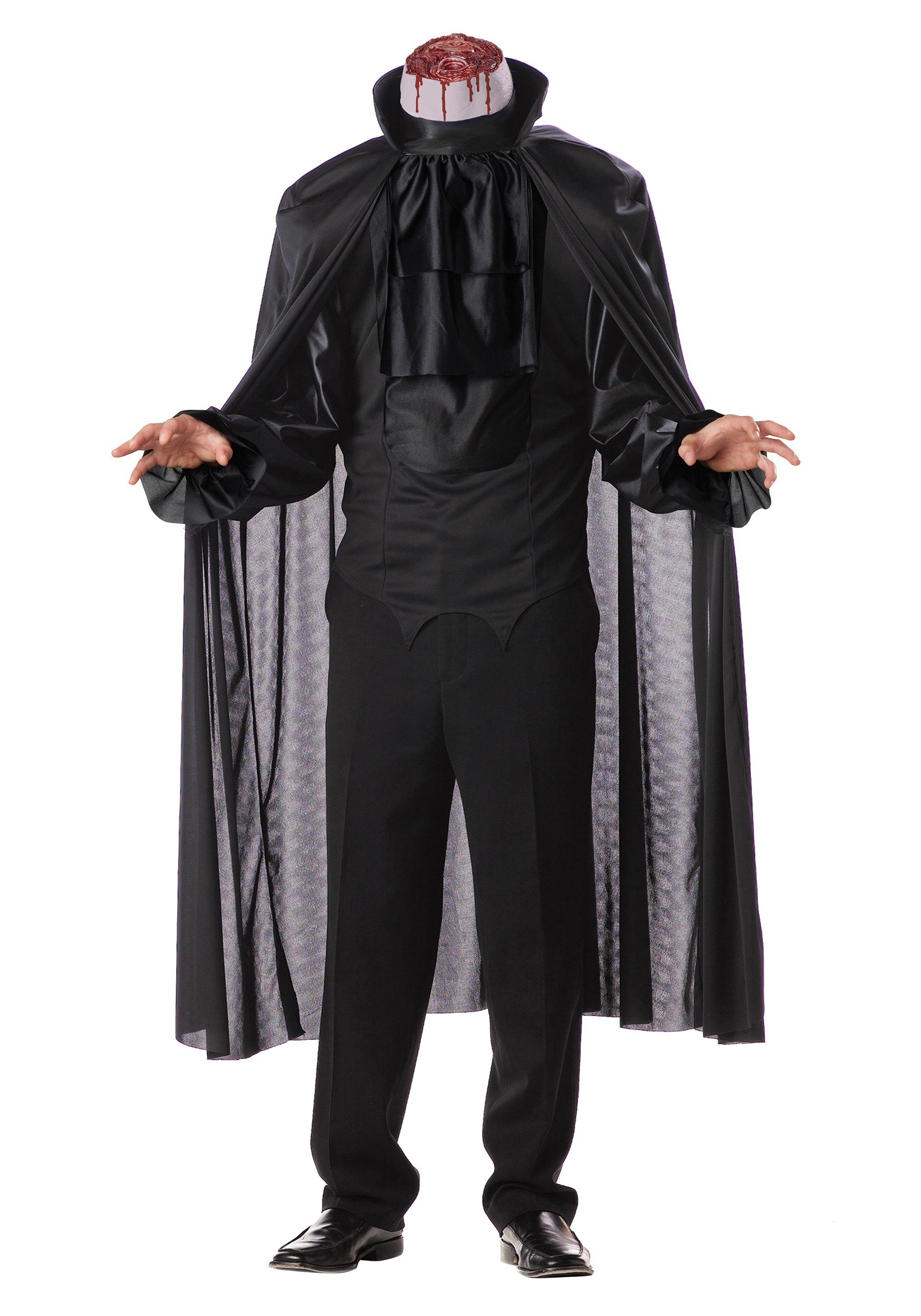The image depicts a costume designed to represent a headless character, likely inspired by the Headless Horseman or a headless vampire. The figure is dressed entirely in black, with a classic, old-timey style that includes a black suit, pants, and shiny formal shoes. The costume also features a luxurious silk cape, black on the outside with a light gray lining adorned with a subtle design. Around the neck area, there is a detailed prosthetic showing a severed, bloody neck with visible bone, complemented by a black ruffled collar. The headless figure appears to be in a menacing stance, with both arms partially extended downward, as if poised to attack.